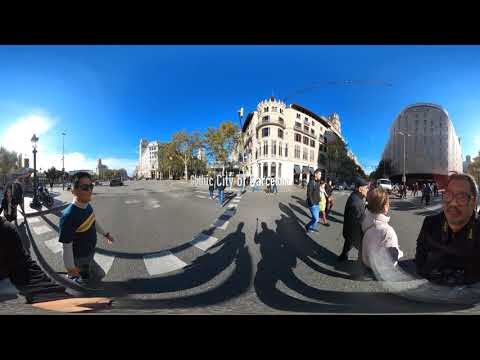The image captures a dynamic street scene in Barcelona, Spain, showcasing a prominent blue sky and towering white buildings adorned with numerous windows. The photo is taken with a convex lens, creating a distinctive curvature that makes the ground and elements like crosswalks bend towards the center. In the middle of the image, partially overlapping the buildings, there is text that likely reads "Public City of Barcelona" or "Gothic City of Barcelona," though it's somewhat difficult to make out due to distortion.

On the street, the asphalt glistens a gray hue, punctuated by distorted crosswalks and shadows of pedestrians that also curve upwards. On the right side, a potential photographer in a black shirt and glasses is noticeable, possibly taking the photo in a panoramic style, giving the impression of a selfie. Nearby, another individual stands with their back to the viewer, wearing a white jacket. To the left, a man clad in a blue shirt with yellow stripes and sunglasses is visible, along with his arched shadow.

The scene is teeming with activity, capturing multiple people traversing both crosswalks and sidewalks. Further enriching the background, white buildings with many floors line the vista, complemented by blue skies speckled with distant clouds. There are street posts with lanterns on the left side, alongside a truck and several streetlights. Additionally, some trees and parked cars are present, adding to the intricacy of this bustling urban snapshot.